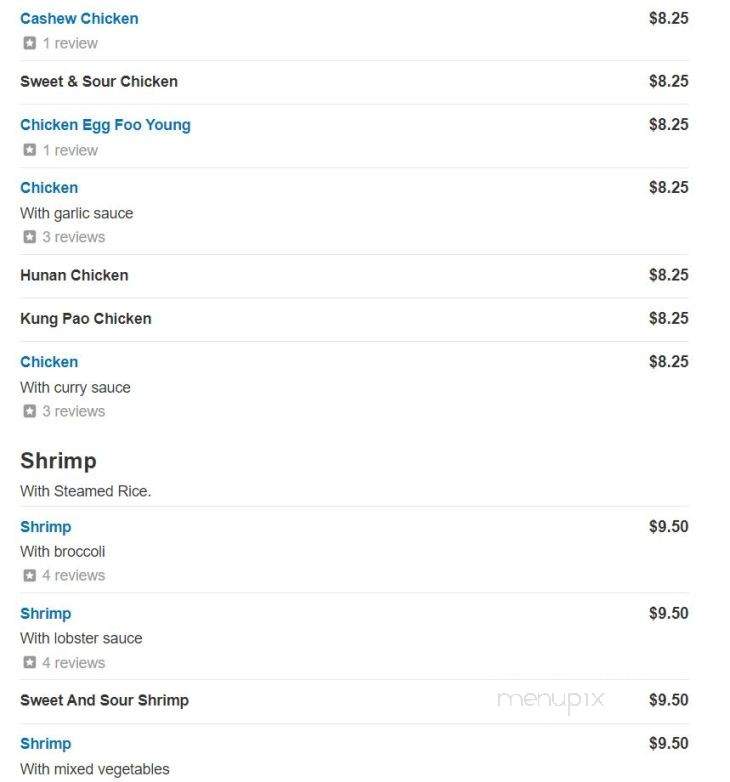This is a detailed screenshot of a restaurant menu featuring various chicken and shrimp dishes, each accompanied by pricing and customer reviews.

At the top of the menu, "Cashew Chicken" is highlighted in blue with one star review, priced at $8.25. Following this, "Sweet and Sour Chicken" is listed in black, also priced at $8.25. Next is "Chicken Egg Foo Young," written in blue, with one star review and an $8.25 price tag. Further down, "Chicken with Garlic Sauce" is shown in blue with three reviews, priced at $8.25. 

"Hunan Chicken" (spelled as H-U-N-A-N) is next, priced similarly at $8.25. Then we have "Kung Pao Chicken" (spelled as K-U-N-G-P-A-O), also costing $8.25. Another dish, "Chicken with Curry Sauce," appears in blue with three reviews, at $8.25.

The menu then transitions to shrimp dishes under the heading "Shrimp with Steamed Rice," though no price is provided for the overall category. The first item is "Shrimp with Broccoli," written in blue, priced at $9.50, with four reviews. "Shrimp with Lobster Sauce," following the same pricing and reviews, also costs $9.50 and has four reviews. Lastly, "Sweet and Sour Shrimp" is noted as a "Menu Pick" (spelled M-E-N-U-P-I-X), priced at $9.50. Below this, "Shrimp with Mixed Vegetables" appears in blue, similarly priced at $9.50.